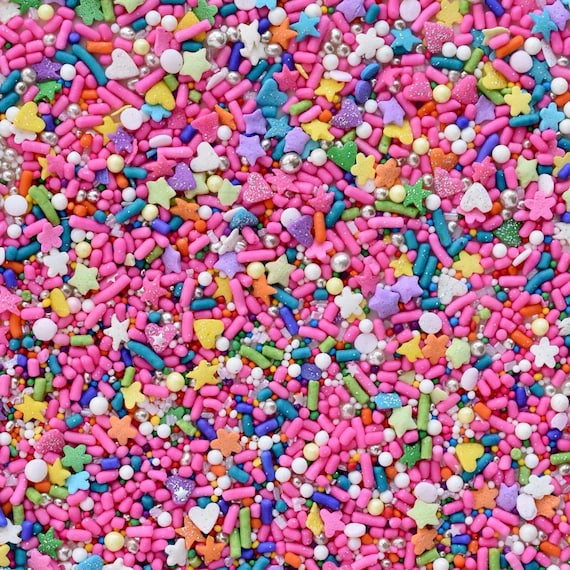This photograph captures an array of vibrant and colorful cake or cupcake sprinkles laid out flat. Dominating the image are hot pink, rod-shaped sprinkles, interspersed with rod-shaped sprinkles in purple and yellow hues. Other notable sprinkles include white and silver pearls, variously colored stars in shades like light green, light yellow, blue, purple, and orange, as well as green stars in multiple shapes. The heart-shaped sprinkles add to the diversity, coming in pink, white, yellow, and blue. Additionally, tiny, multicolored round sprinkles and some flower-shaped ones enhance the multicolored, predominantly pastel palette. The entire scene is brightly lit, highlighting the shiny, candy-colored sprinkles and creating a visually appealing, cheerful image.